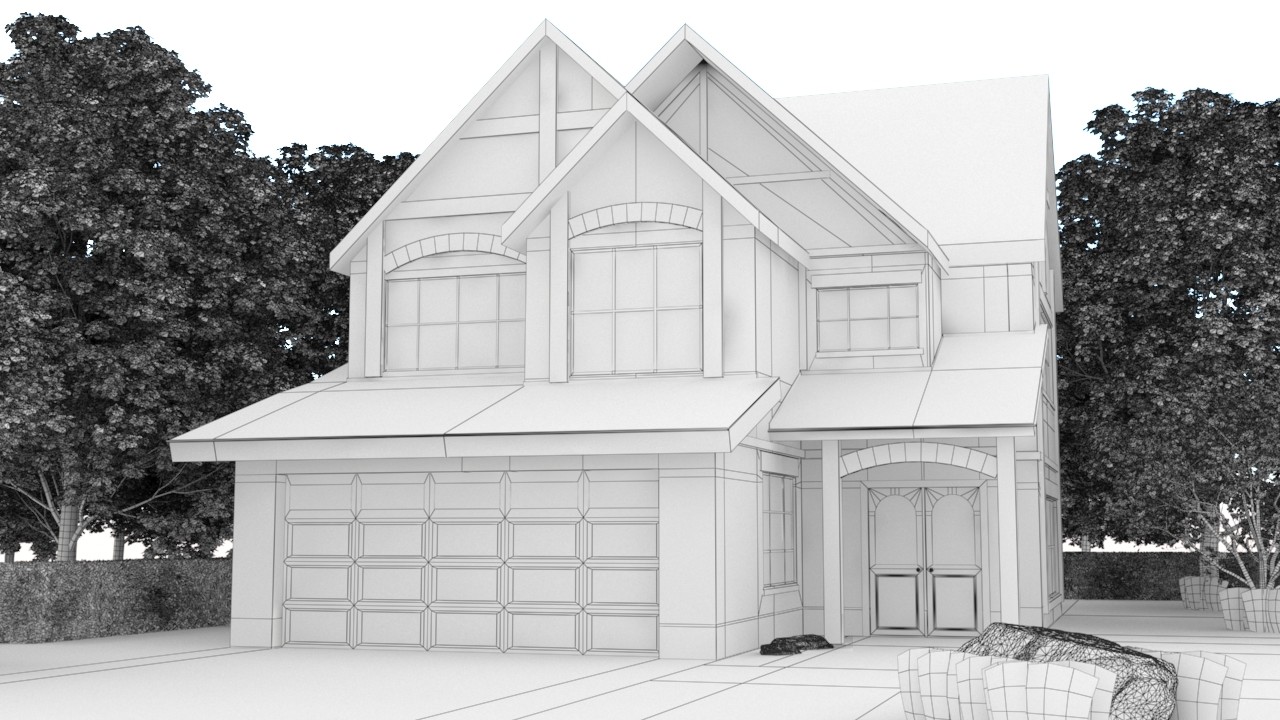This rectangular image, approximately six inches wide and three inches tall, portrays an artist's 3D rendition of a house in black and white. The top third of the image shows a plain white background resembling the sky, devoid of any corners or borders. The ground appears to have a white surface with black grid lines intersecting it. Flanking the sides of the image are gray-colored trees and low-lying hedges, giving a sense of scale and depth. The centrally positioned house model exhibits detailed structural elements in black lines that define the crossbeams, roofs, and arches. The house itself is two-story, featuring a large two-car garage on the left side. A driveway leads up to this garage, and there are two windows with small arches above them situated over the garage door. To the right of the garage, recessed slightly with an overhanging roof, is the main entrance highlighted by a series of pillars and a prominent archway. This archway leads to double French-style doors. The second floor of the house displays three dormers, each with distinct slopes facing forward, while another slope extends backward, rounding out the roof design. The area surrounding the house includes carefully placed trees in pots and a small patio area in the bottom right-hand corner, adding to the lifelike feel of the model.